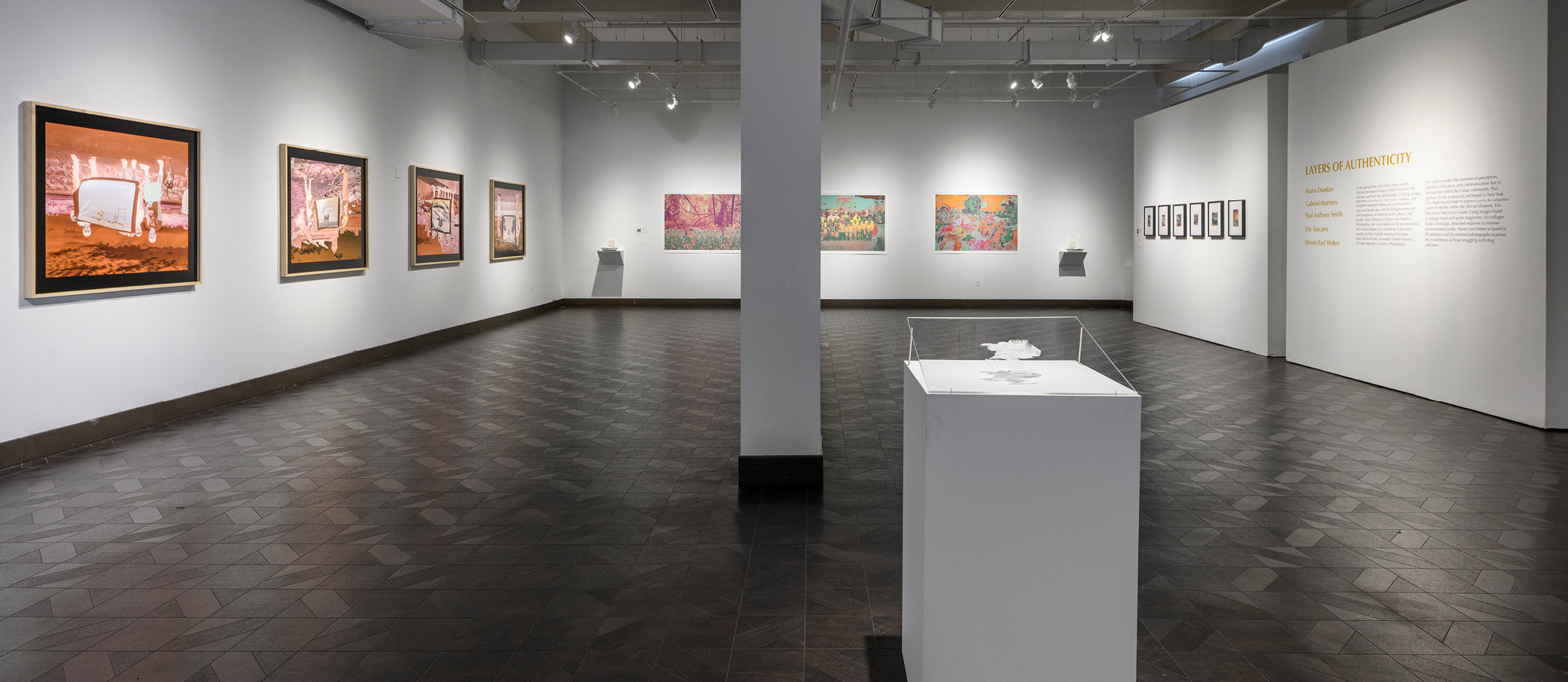The photograph captures the interior of a modern art museum. Central to the image is a white display case atop a white pedestal, containing a small, indistinct 3D object. The museum features three prominently visible walls adorned with various artworks. On the left wall, four sepia-toned and orange-hued modern art pieces are displayed. The back wall showcases three vibrant paintings, rich in colors like orange and teal, likely depicting landscapes. The right wall features six small framed artworks and a section of text headed "Layers of Authenticity", though the finer details of the text are unreadable at this distance. A white column descends from the ceiling near the center, and the dark patterned floor contrasts with the clean white walls and the track lighting overhead, contributing to the contemporary atmosphere of the space.